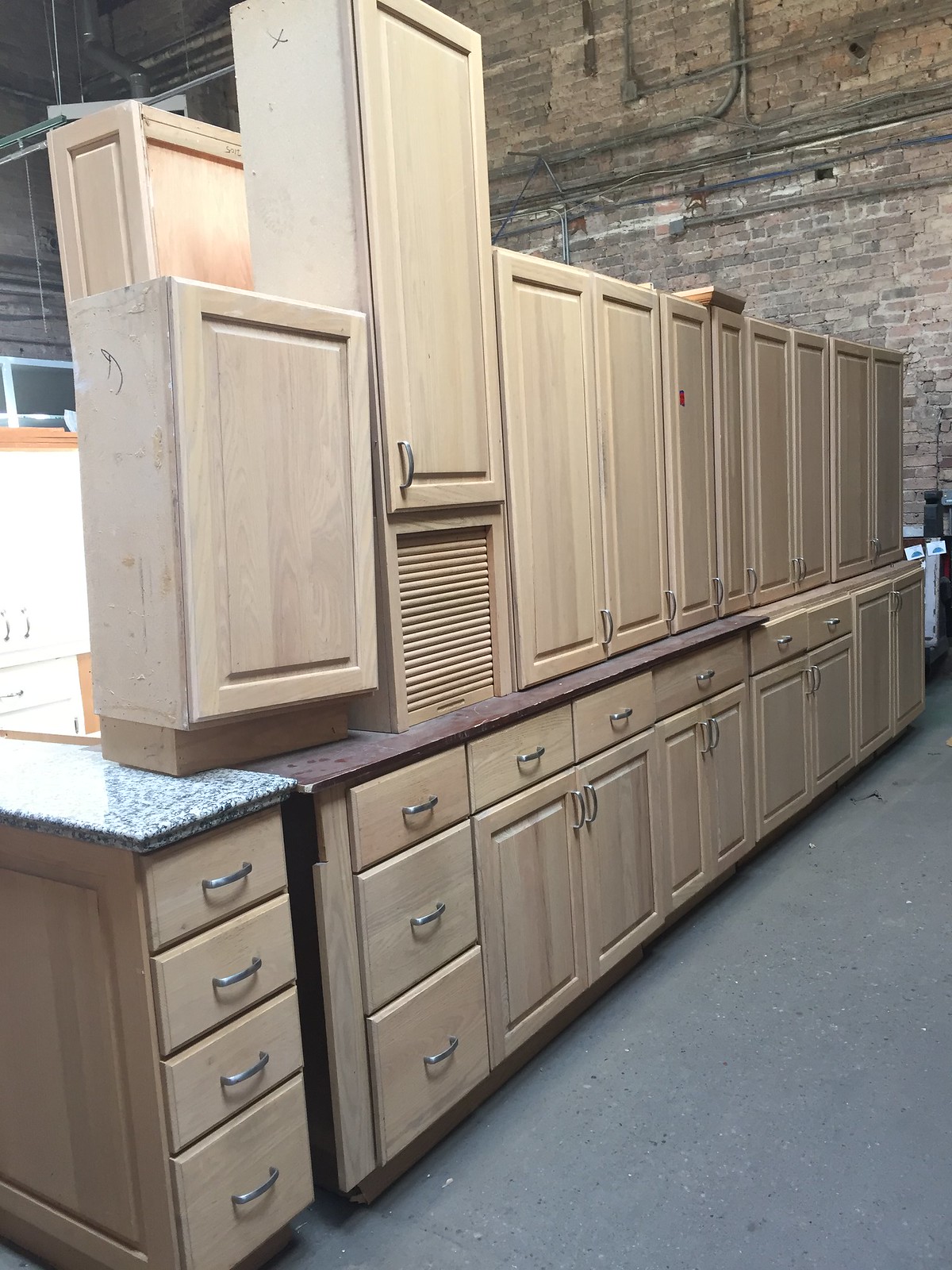This color portrait photograph showcases a neatly arranged set of kitchen cabinets stored in what appears to be a workshop or warehouse. The image features both upper and lower cabinets, all constructed from the same light-colored wood. The lower cabinets include several units: two with drawers, three with a single drawer over doors, and one with a pair of double doors. One unit notably lacks hardware. The upper cabinets all have solid wood doors. A unique feature is a small appliance garage integrated into the set. A section of granite countertop is visible, placed over a single lower drawer unit. The cabinets are outfitted with uniform silver handles—horizontal for the drawers and vertical for the doors. They are situated in a room with a high, light-colored brick wall and a concrete floor, adding a utilitarian backdrop to this organized display.